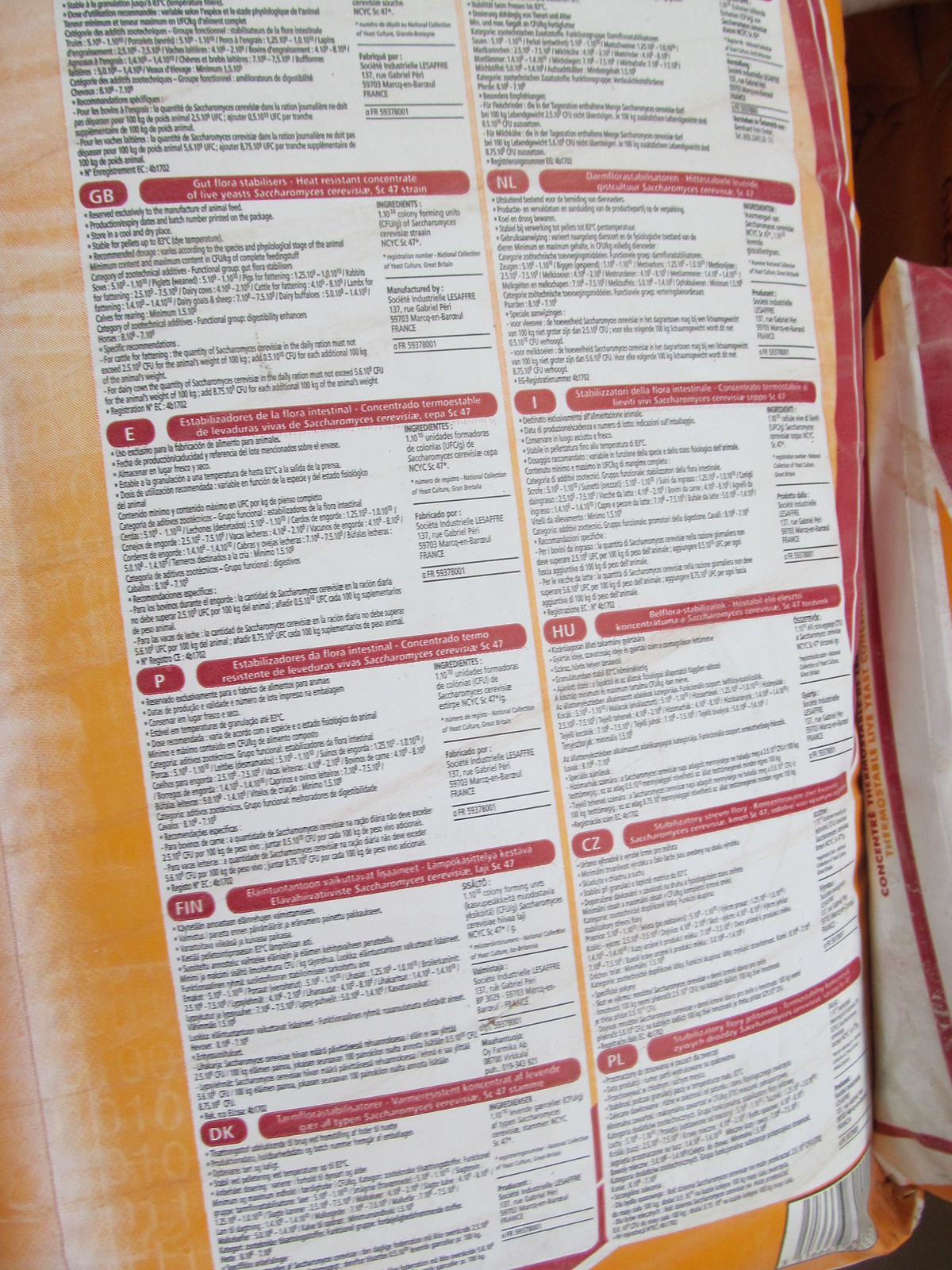The image showcases a large, orange bag primarily occupied by an extensive white label adorned with red banners. The label is densely packed with multilingual information, detailing the contents and usage of a gut flora stabilizer that includes a heat-resistant concentrate of live yeast. Also present on the label are ingredient specifics and manufacturing details, including the marking "GB." Various languages are represented on the label, with potential inclusions of Finnish, Czech, Hungarian, Spanish, and Italian, repeating the same descriptions. At the bottom right-hand corner of the image, a barcode is visible, enhancing the informational aspect of the packaging.